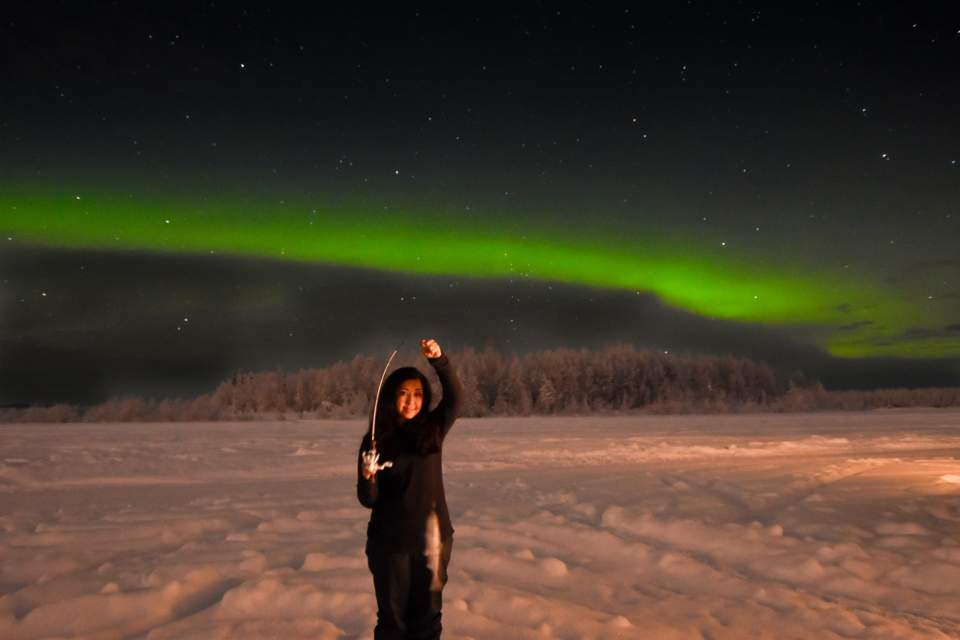A woman stands at the center of a snowy landscape, framed by a backdrop of frost-covered ground and brown trees. The night sky above is a deep, inky black, adorned with a multitude of stars. Dominating the sky is a mesmerizing display of the northern lights—a vivid, neon green aurora that stretches horizontally across, almost resembling a science fiction phenomenon. The green light is contrasted by a gray section of the sky beneath it. The woman, dressed in black, grasps an object that looks like a fishing rod with a uniquely shaped long, skinny end and a broader base. With one hand holding this rod and the other raised above her head, she strikes a dramatic pose. The scene is illuminated just enough to highlight tire tracks imprinted in the snow, adding to the surreal and almost digitally enhanced ambiance of the image.